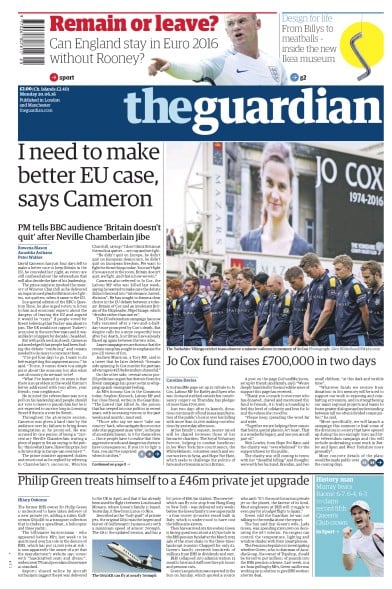This image is a screenshot of the front page of The Guardian newspaper. 

At the top, a prominent headline reads, "Remain or Leave," followed by another headline in bold black text: "Can England stay in Euro 2016 without Rooney?" Next to this headline, a barcode runs vertically up the left side. To the right, there is an image of a soccer player, possibly in his 30s, with fair skin wearing a white soccer jersey. His right arm is outstretched, pointing to the side.

Below, another headline in blue text reads, "Designed for Life," followed by "For Billy's to meatballs inside the new" (unable to decipher the rest). This section includes an image of a gray, silver-like pole shaped in an 'S' over a yellow circle.

The Guardian's banner runs across the page, with a top headline stating, "I need to make better EU cases – Cameron." The subhead adds, "PM tells BBC audience he doesn’t quit after Neville Chamberlain jibe."

To the right, there is a significant image of several men wearing black uniforms with yellow stripes. Below this, a billboard for Joe Cox is visible, featuring an image of Joe Cox standing in front of a house. The headline beneath this image announces, "Joe Cox fund raises seven hundred thousand pounds in two days."